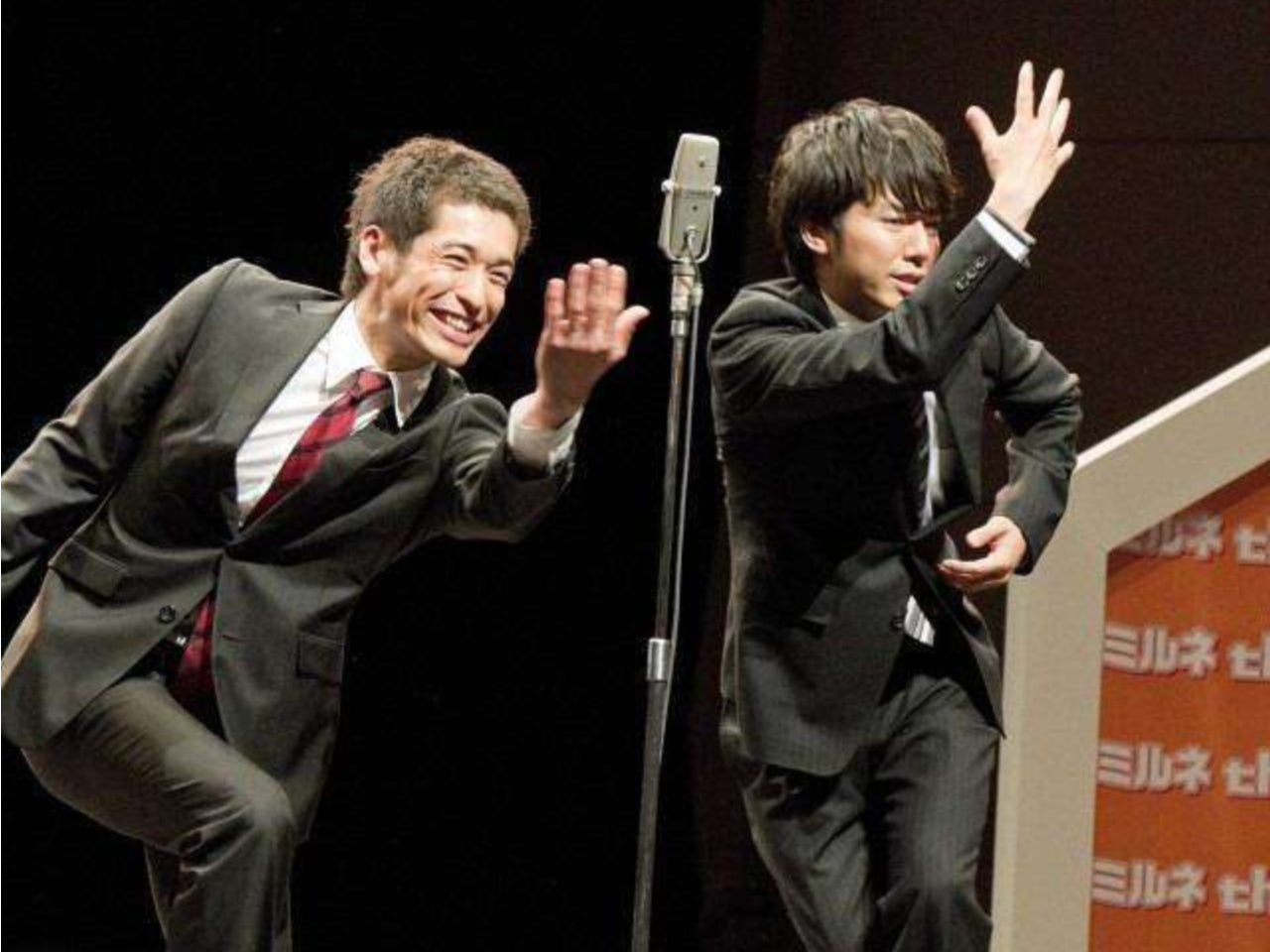This close-up photograph captures two young Asian men, likely Japanese, energetically performing on stage. Both are attired in dark suits with white button-up shirts and ties; the man on the left sports a red plaid tie and has short brown choppy hair, while the man on the right, with longer shaggy black hair, wears a dark tie and pinstripe pants. They are mid-dance, each with arms extended and expressive hand gestures. The man on the left has his left hand stretched out, beckoning with a big smile, while the man on the right has his right arm raised and his left arm bent inward, suggesting he is carrying something tall. Positioned between them is a floor microphone, indicating they might be singing as well. The stage backdrop is black, and there is a partially visible sign with an orange area and white text to the right, framed in beige. This striking image emphasizes their dynamic performance and joyful expressions.